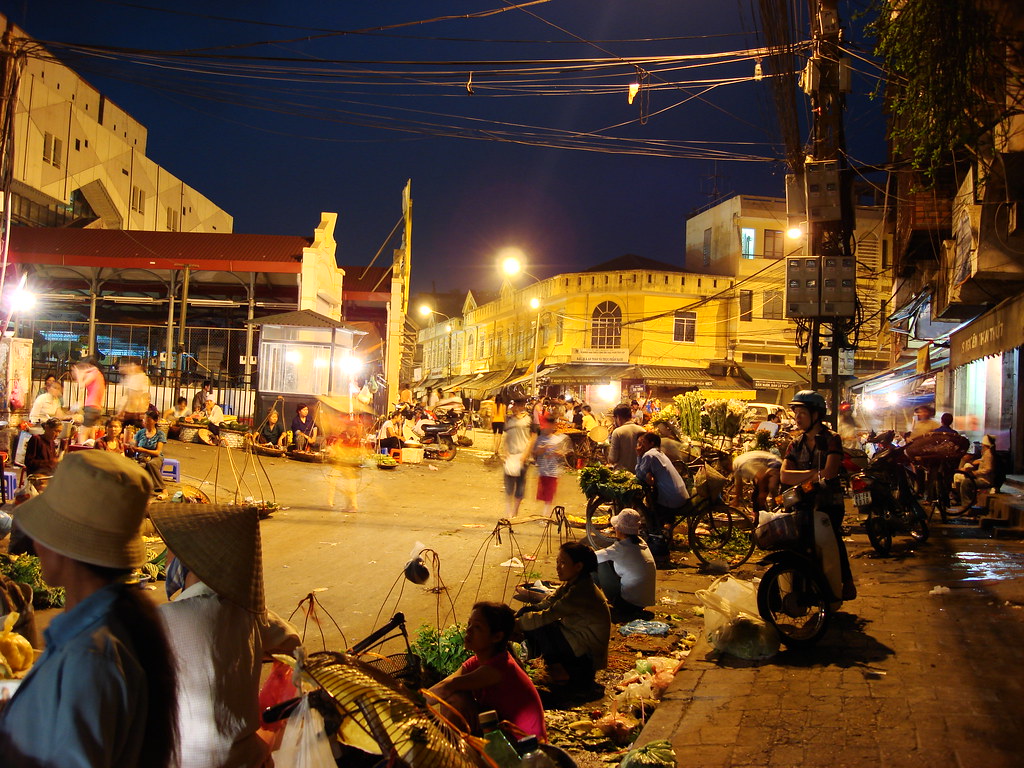The photograph captures a bustling night market in Ho Chi Minh City, Hanoi, Vietnam, taken in landscape orientation. The image vividly portrays the scene under the night sky, enveloped in the warm yellow glow from various streetlights and floodlights. This realism-style photograph is rich in detail, revealing a crowded street devoid of cars but filled with people, vendors, and scooters.

In the center of the market, an artist is seen performing a magic trick, attracting the attention of many passersby. Surrounding this central point, a plethora of vegetable vendors sit on the ground, bicycles, or carts, offering their goods to the numerous shoppers walking around. The streets are lined with open shops and colorful structures, such as one with a distinctive red roof on the left side, where people are seated on the curb. Sidewalks on either side of the street are crowded with vendors using various instruments for cooking and entertainment, contributing to the vibrant, chaotic ambiance.

Notable details include a large telephone pole on the right sidewalk, bristling with an array of wires stretching across the street. The atmosphere is dense and lively, capturing the essence of a typical night in a street market of the region, with the hustle and bustle of vendors and customers alike.